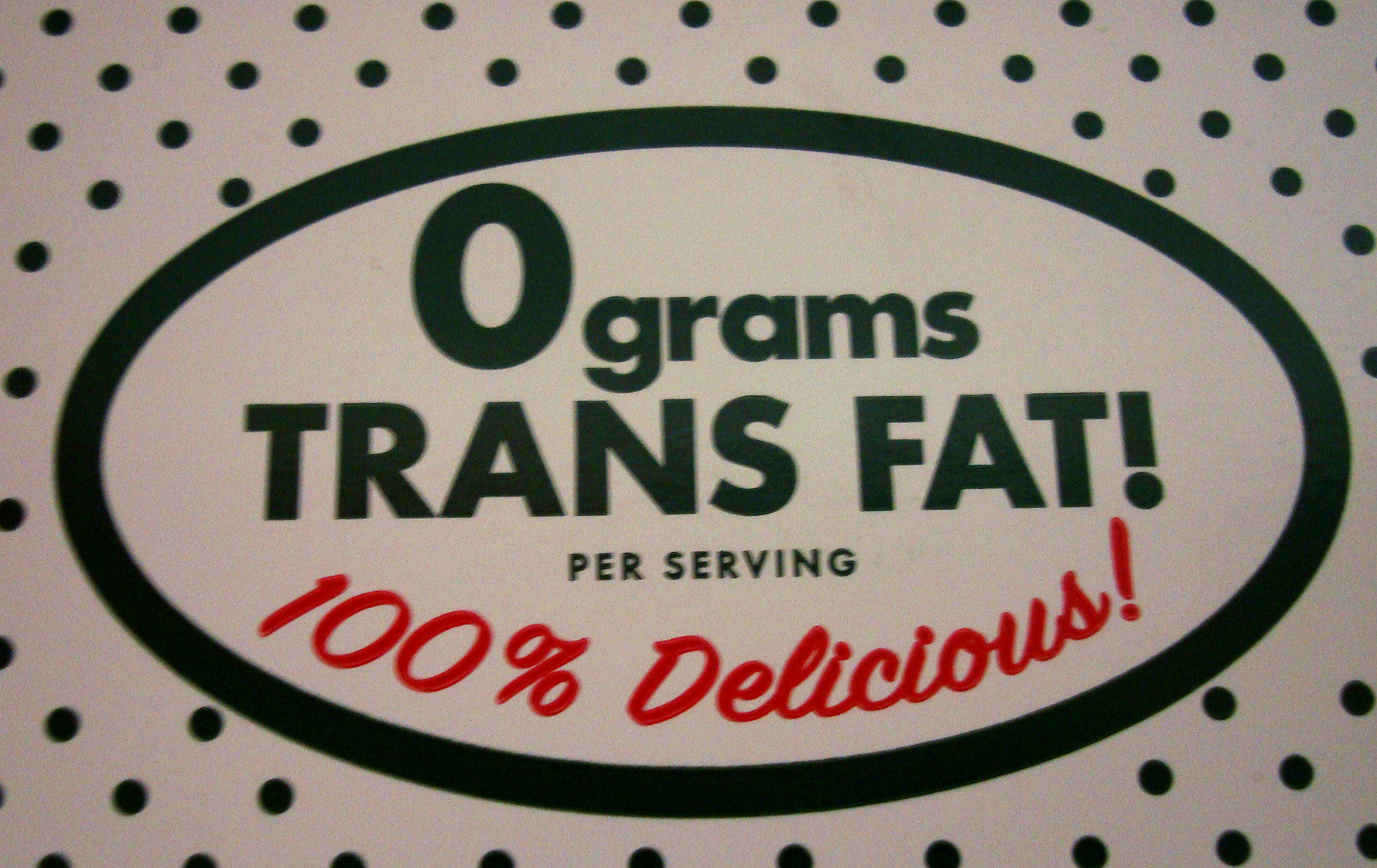The close-up photograph displays an intricately designed label from a food product, prominently featuring nutritional information. The label is set on a white background adorned with densely spaced, almost black dark green polka dots. These dots surround an elongated oval shape with a thick black outline. Inside the oval, in bold black text, it prominently states "ZERO grams" with the numeral "ZERO" notably larger and outlined in black. Beneath this, the text "TRANS FAT!" is capitalized and followed by an exclamation mark. Further down, but still centered, it reads "per serving" in smaller black text. Paralleling the oval’s outline in red cursive text, it proclaims "100% delicious!" with the word "delicious" styled in a flowing, italic script. The overall design suggests an appealing advertisement, emphasizing the absence of trans fat and the promised delightful taste of the product, reminiscent of a Krispy Kreme box.